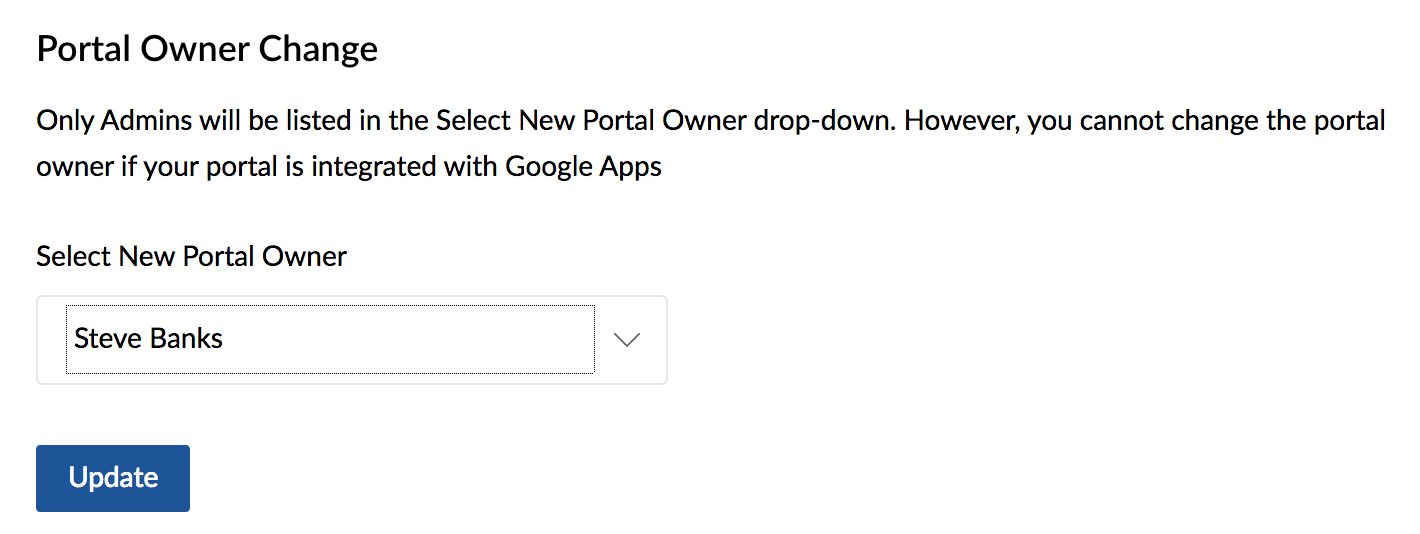The image depicts a webpage interface from a settings section, likely related to managing administrative controls. The top of the interface displays a header that reads "Portal Owner Change." Below this, instructional text indicates that only administrators are listed in the "Select New Portal Owner" drop-down menu, with a caveat that changes to the portal owner cannot be made if the portal is integrated with Google Apps.

Beneath this text, there is a white drop-down text box with a black border, currently displaying the name "Steve Banks" in black text. Adjacent to this box is a downward-facing arrow, suggesting that clicking it will reveal more options. Below the drop-down, prominently centered, is a blue button labeled "Update" in white text, which presumably, when clicked, will finalize the change of the portal owner.

The interface is set against a clean white background with predominantly black text for clarity. The structured layout and standard web design elements confirm it is from a webpage's settings section, intended for administrative users to manage portal ownership settings.